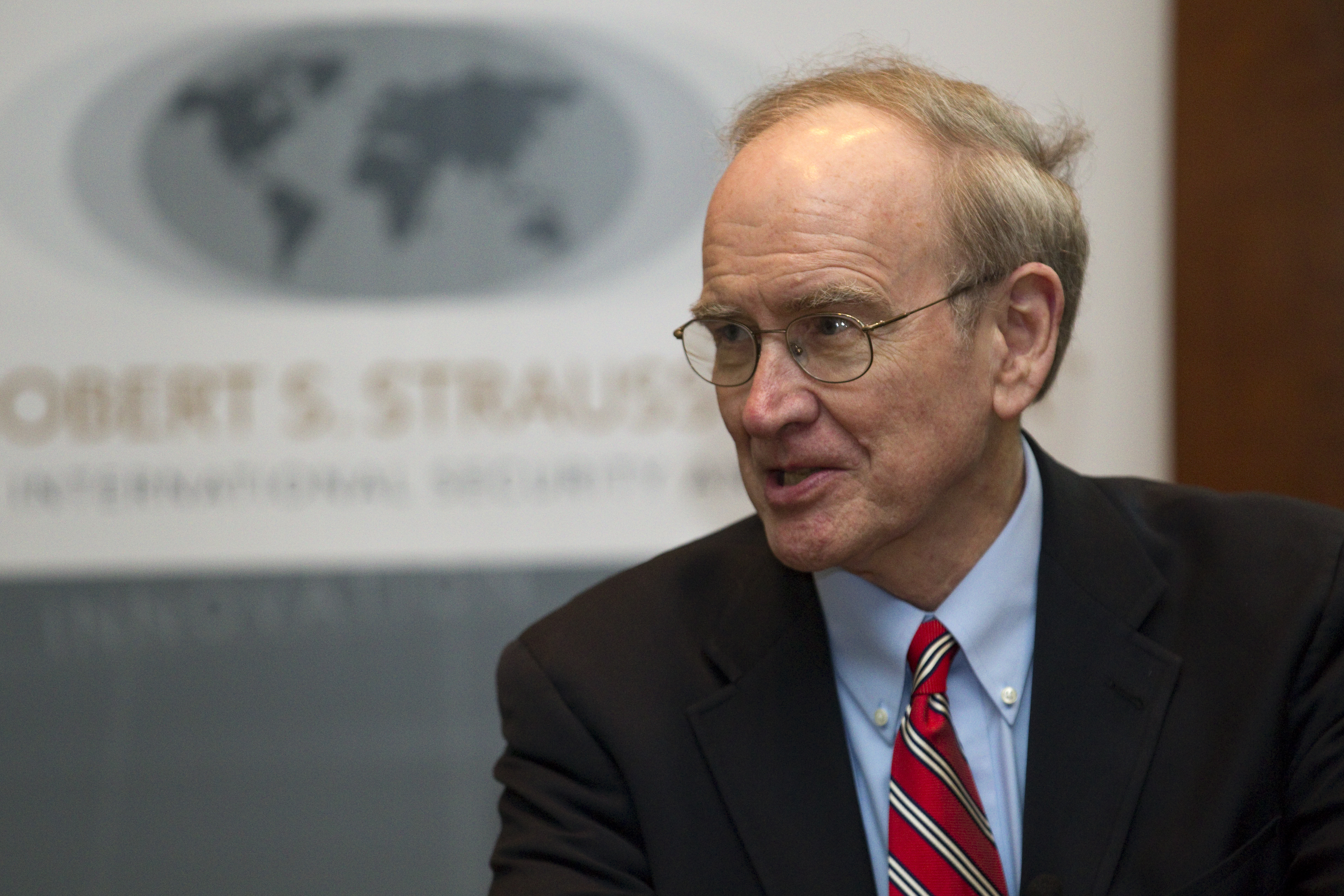The image appears to capture a formal event or business meeting setting. In the background, there's a wall adorned with a blurred banner that partially reads "obert s Strauss." The banner features an oval-shaped depiction of the planet, showcasing different continents with a gray earth and darker shadows marking the landmasses. The banner is positioned more towards the left side of the image.

The focus of the picture is an older gentleman seated on the right-hand side. He has a balding head with a comb-over parted to the left, sporting hair that appears to be a mix of gray, brown, and blonde. He wears thin eyeglasses and seems to be engaging in a conversation with someone off-camera. His expression is mostly serious with a hint of contentment. He is dressed in a dark gray blazer, a blue button-down shirt, and a red tie adorned with white and black diagonal stripes.